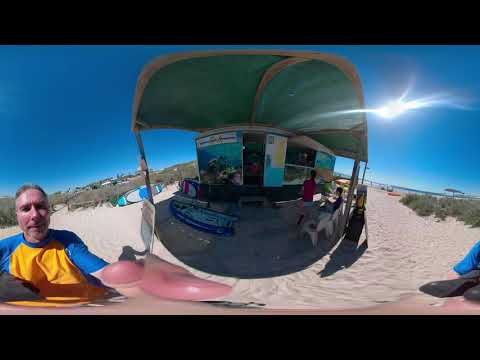The panoramic beachside image features a central hut with a green canopy, distorted by a fisheye lens. The hut, sitting on rippled beige sand, has a service window where people are standing to order, and a person is seen sitting at one of the benches or tables in front of it. The hut is adorned with pictures around the window that are too blurry to identify clearly. Surrounding the hut are some green shrubs, and in the distant background, there is a bridge-like structure and an umbrella. The sky above stretches in a bright aqua or teal hue with a distorted sun to the right. To the bottom left, the probable photographer, a middle-aged white man with some gray hair, a possible beard, and wearing a gold and sky-blue short-sleeved t-shirt, is partially visible. His arm appears on the right-hand frame while the rest of his body is seen on the left side of the image.